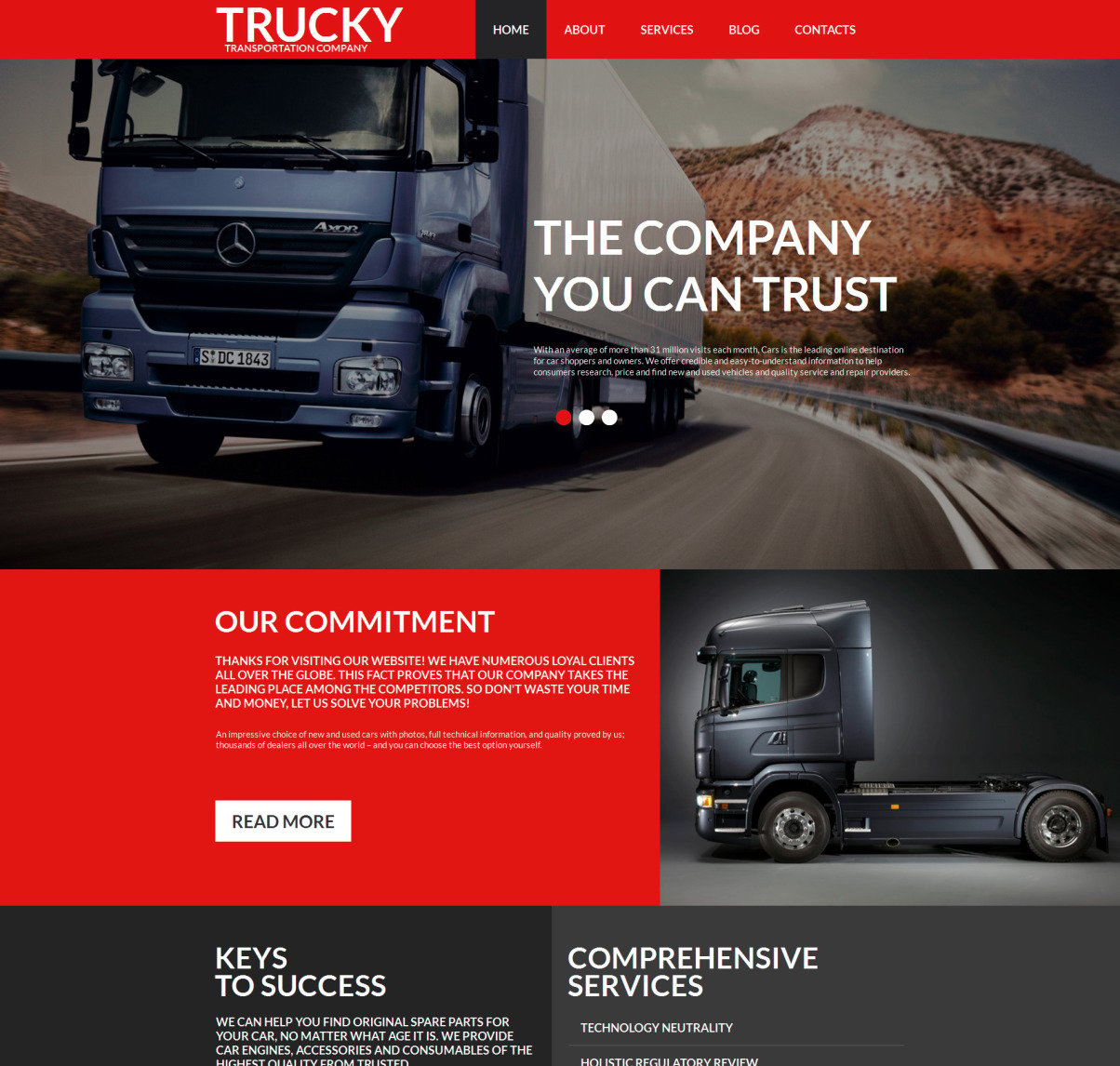This image is an advertisement for the Truckee Transportation Company. At the top, there is a navigation menu within a red rectangular box, featuring links labeled "Home," "About," "Services," "Blog," and "Contacts." Below this, a high-resolution picture showcases one of Truckee's trucks—a blue Mercedes with a flat front windshield, indicating a cab-over-engine design.

In the main section, a red box highlights the company's mission with the text: "Our Commitment, The Company You Can Trust." The accompanying message reads: "Thanks for visiting our website. We have numerous loyal clients all over the globe. This fact proves that our company takes the leading place among competitors. So don't waste your time and money. Let us solve your problems." A "Read More" link is provided for further information.

Additionally, a black box titled "The Keys to Success" explains the company's value proposition: "We can help you find original spare parts for your car, no matter what age it is. We provide car engines, accessories, and consumables of the highest quality from trusted dealers." Finally, a gray box with the title "Comprehensive Services" partially visible states "Technology Neutrality." 

The advertisement intends to highlight Truckee Transportation Company's reliability, global client base, and extensive services.